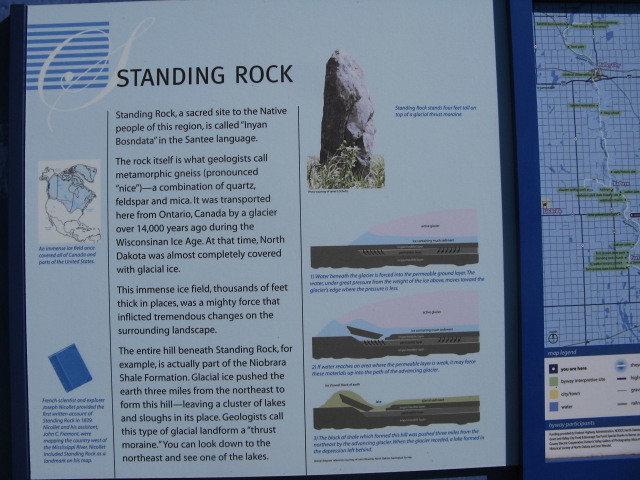The image depicts an informative graphic, likely from a museum display, characterized by a bluish hue. The display is split across two pages, with the right-hand side partially cut off. The left page prominently features the title "Standing Rock," alongside a photograph of the rock itself. Below this image is a caption detailing its significance as a sacred site for the native people of the region, known in the Santee language as Inyan Boznadata. The rock, identified by geologists as metamorphic gneiss (pronounced 'nice'), comprises quartz, feldspar, and mica. It was transported from Ontario, Canada, to its current location over 14,000 years ago during the Wisconsin Ice Age, when North Dakota was enveloped by a massive glacier. This ice sheet, thousands of feet thick, dramatically reshaped the landscape, forming what is known as a thrust moraine. The entire hill beneath Standing Rock is part of the Niobrara Shale Formation, displaced by the glacier's incredible force. Additional visuals include a United States and Canada map with diagrams illustrating the glacier's movement and its resultant landforms. There's also a photograph of the rock from different angles and a smaller image showing how the rock split over time, accompanied by brief captions that are somewhat difficult to read.